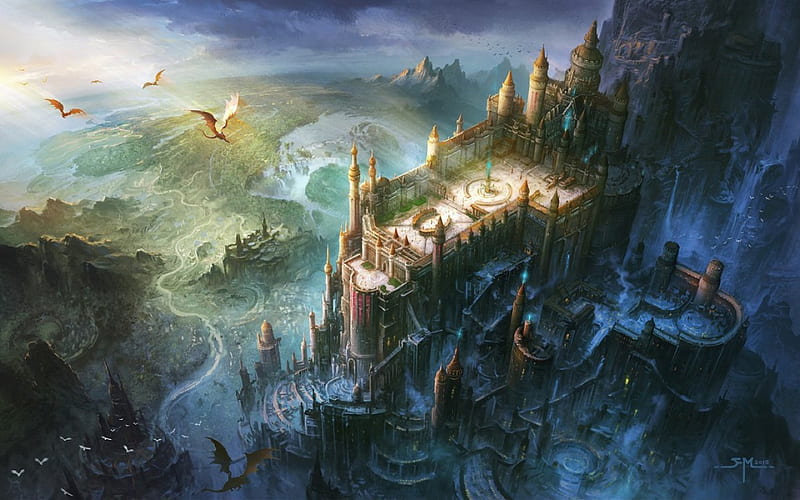This highly detailed and surreal artwork depicts a fantastical and futuristic multilevel castle with numerous turrets, courtyards, and intricate architectural elements, branching out in a grandiose manner. The castle, rendered in varied tones of beige and brown, stands imposingly against a backdrop of mountains with small pointed peaks. To its left, a possible moat or body of water reflects the structure's majesty. The scene is populated by numerous flying creatures, including three to four large, beige and brown bird-like creatures with massive wings in the upper left, and about ten smaller white birds in the bottom left.

Further enhancing the surreal atmosphere, the background includes tall, dark structures resembling mountains or additional fortifications. The sky, predominantly situated in the upper half of the image, appears dynamic with these creatures soaring through it. Adding a touch of mystery, there is a semi-legible artist's signature in the left part of the image, featuring prominent letters "F" and "M," hinting at its origin.

Overall, the image exudes a dark yet intriguing aura, with a style that mixes medieval and futuristic elements, reminiscent of video game art, and evokes a sense of otherworldly adventure.